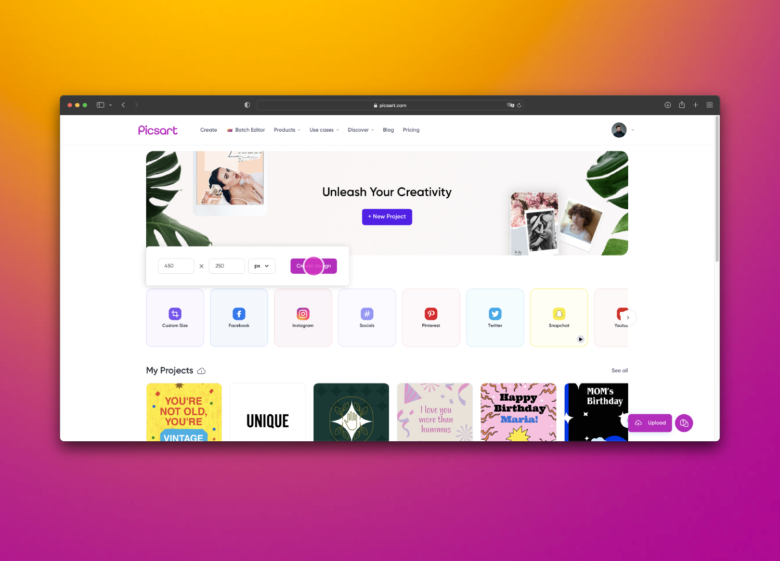The image depicts a vibrant and colorful website displayed on a computer screen, set against a dynamic screensaver with shades of orange, pink, light pink, and light orange. The website, named "Picsort," prominently features its title flanked by palm leaf illustrations on both the left and right sides of the screen, which are vertically white.

At the top of the screen, the website's title is accompanied by the familiar red, gold, and green buttons of a computer interface. On the right side, standard computer icons are visible. In the center of the page, in large, bold black letters, the phrase "Unleash Your Creativity" stands out, inviting users to explore the site's features.

Beneath this slogan, a purple clickable box is shown, accompanied by an image of a girl with her head tilted back, adorned with makeup, likely signifying the creative possibilities offered by the site. To the right, there are additional images, including one of a girl, one of flowers, and another that appears to depict a girl and a guy.

The central area of the site features three dropdown menus, with various images horizontally aligned beneath them, allowing users to pick from options such as Facebook, Twitter, and Pinterest for sharing their creations.

At the bottom, there is a section labeled "My Projects," showcasing several distinct designs: 

1. "You're Not Old, You're Vintage" in yellow.
2. "Unique" on a white background with black letters.
3. A black background featuring a white star.
4. A festive design with the text "I Love You," featuring party hats and banners.
5. "Happy Birthday, Maria" positioned second to the last.
6. The final project titled "Mom, Birthday," accompanied by a purple box. 

This detailed layout emphasizes the website's focus on creativity and custom project creation, offering a variety of templates and sharing options for users.